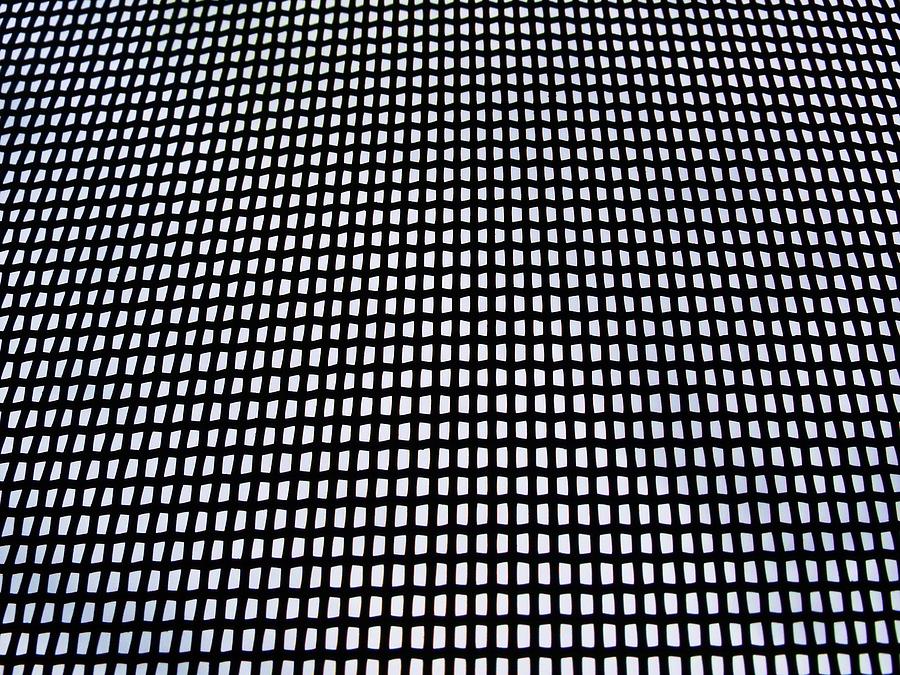The image features a symmetrical, repeating pattern in a rectangular format with all sides measuring equally, giving it a square appearance. The pattern comprises densely packed black lines that intersect to create an array of identical white rectangles or squares. These shapes are arranged in multiple rows and columns, with each white rectangle being slightly taller than it is wide. The pattern extends beyond the edges of the photograph, leaving it ambiguous whether it continues indefinitely or ends at the photograph's boundary. The entire image is filled with this black grid design, forming the illusion of numerous tiny white squares framed by black lines. There are no objects, text, or other colors present, making the image solely black and white. The close-up perspective suggests the possibility of the grid being viewed at a slight angle, contributing to the symmetrical and orderly visual effect, characteristic of graphic design or artwork.